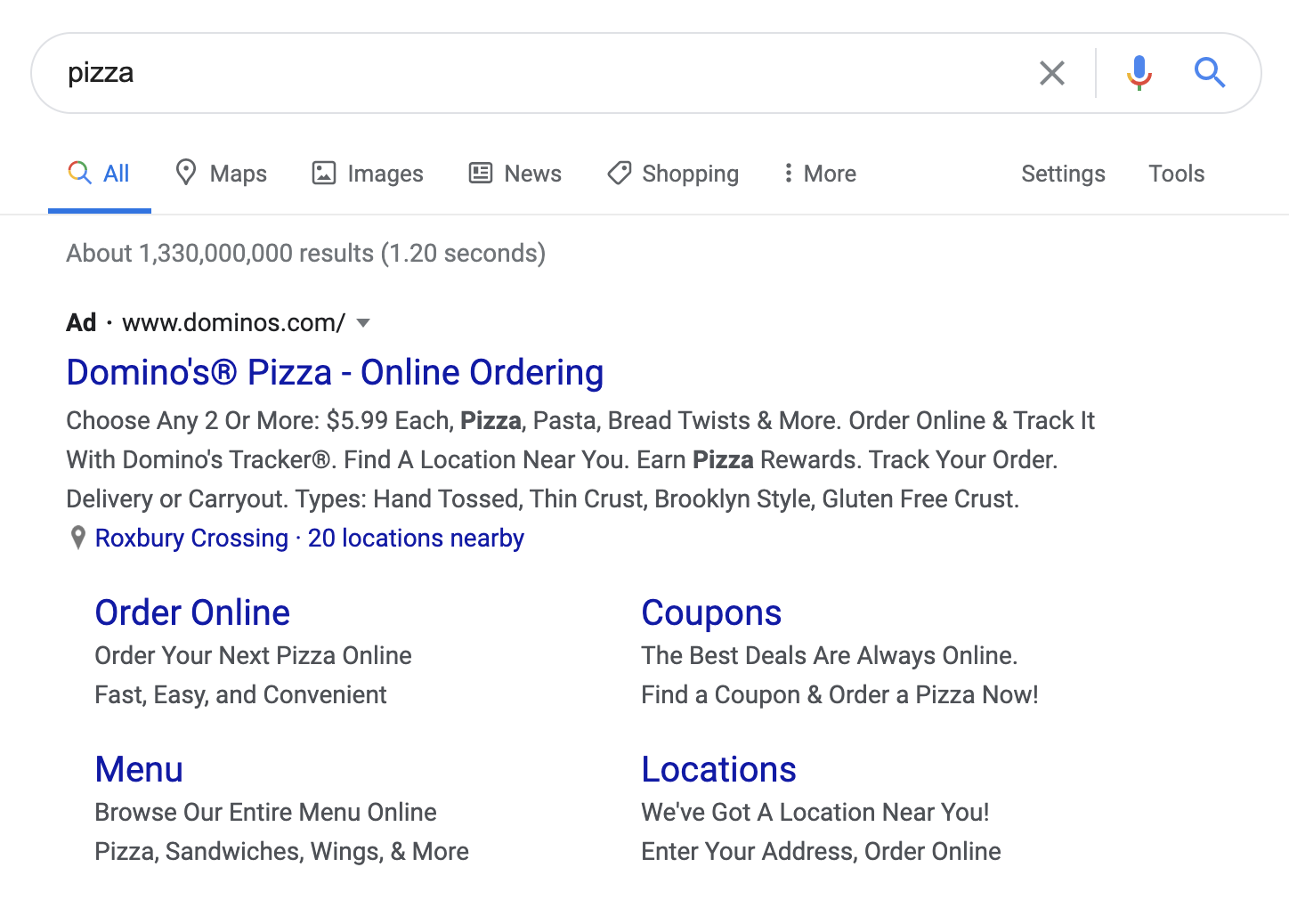The screenshot captures a Google search results page after querying "pizza." At the top, the search term "pizza" is visible in the Google search bar, which also features an 'X' icon to clear the search, a microphone icon for voice search, and a magnifying glass icon to initiate the search. Below the search bar, there's a navigation menu with "All" selected. The menu options include Maps, Images, News, Shopping, and More. On the far right are options for Settings and Tools.

Below this navigation bar is a line separator followed by a message in gray text indicating the number of search results: roughly 1,330,000,000 results found in 1.20 seconds. The first result displayed is an advertisement for Domino's Pizza's online ordering service. This ad includes a brief description of the services offered and notes that there are 20 Domino's locations near Roxbury Crossing.

Beneath the ad are four options related to the Domino's Pizza site: "Order Online" in the top left, "Coupons" in the top right, "Menu" in the bottom left, and "Locations" in the bottom right. Each of these sections includes short descriptions of what users can expect to find if they click on the respective links.